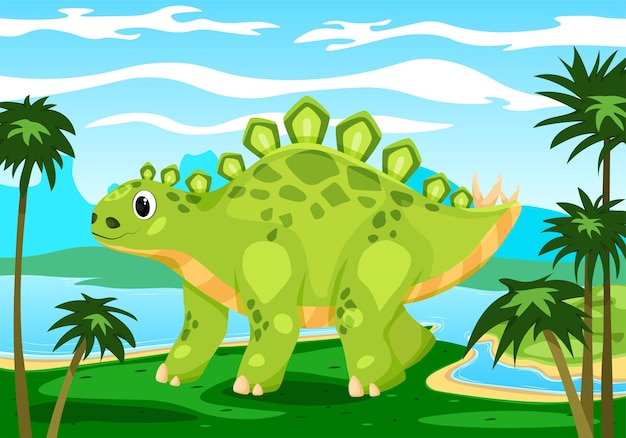This cartoon image features a friendly, large green dinosaur with darker green spots and a yellowish-tan striped underbelly. The dinosaur, which resembles a stegosaurus, has four thick legs, each ending in white nubs that look like blunt claws. The creature's body is adorned with a series of light green to dark green spikes running along its spine from its head to its short, stubby tail. Its smiling face, characterized by a big, expressive black and white eye, adds to its endearing appearance. The dinosaur stands on a grassy expanse with tall, thin palm trees with shaggy green tops on either side in the foreground. Behind the dinosaur, a serene landscape unfolds, featuring a blue river or waterway, a strip of sandy beach, and distant greener land. Above, the sky is a gradient of light blue with scattered white clouds. The scene captures a blend of natural elements, giving it an inviting and cheerful atmosphere.